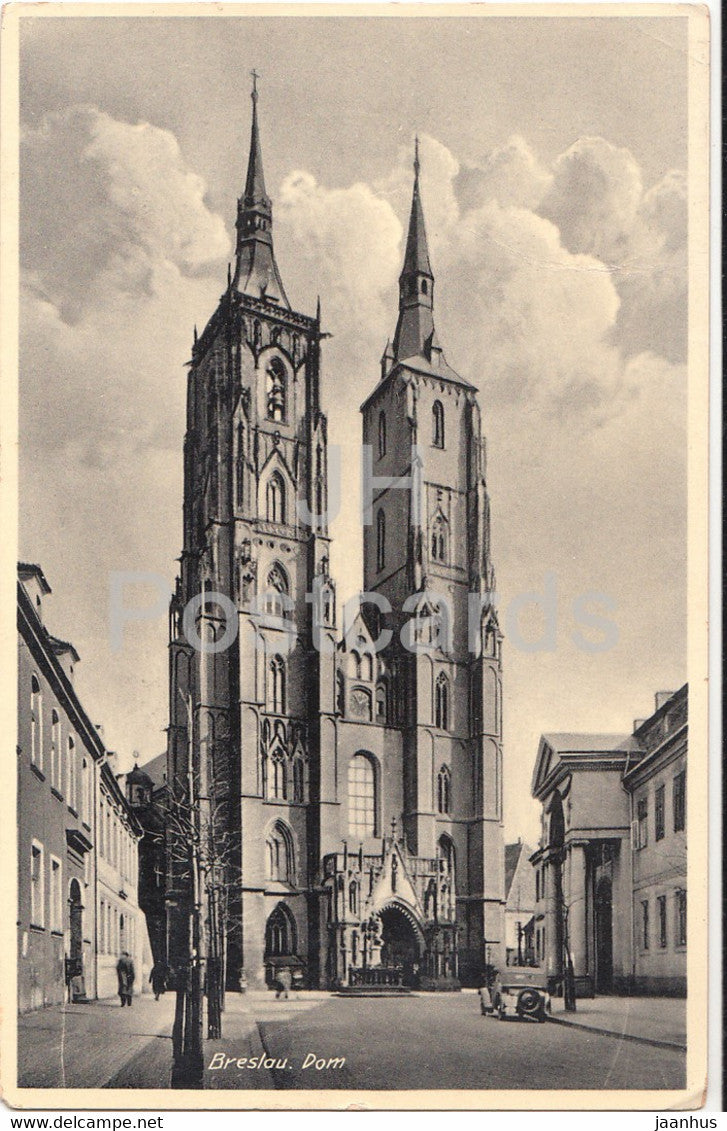This image appears to be an old-time photograph, possibly from a historical catalogue. It features two prominent church spires reaching towards a backdrop of clouds. Across the middle of the photo, there is an illegible watermark that seems to spell "ORTCANDS." At the very bottom of the photo, text reads "WWW.DECLAMPED.NET." In the lower right corner, the name "JAANHUS" is printed. Additionally, written in white on the photograph is the word "BRESLOU." The image shows a street leading directly to the church, with what looks like a courthouse building on the right side and a series of shops on the left.